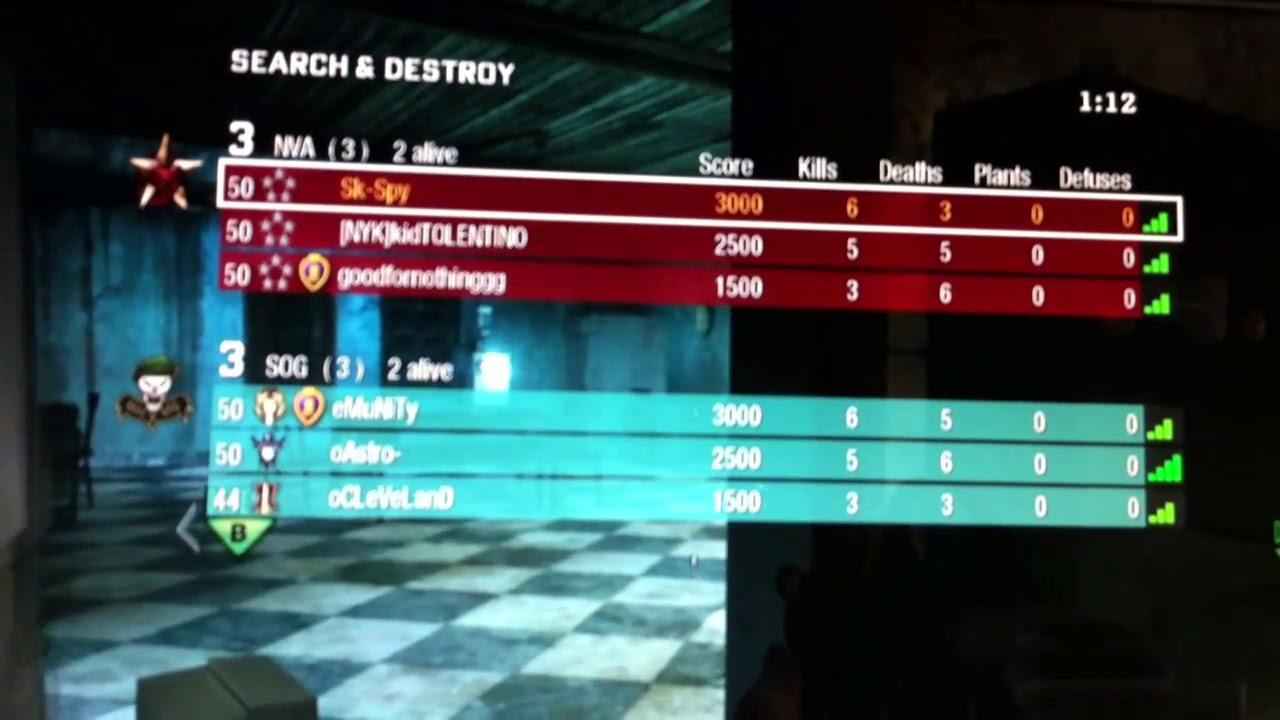The image portrays a screenshot from a competitive video game titled "Search and Destroy." Dominating the scene is a split screen with the top half displaying "SEARCH AND DESTROY" in capital white text against a partially black and checkered background. The top corner to the right shows a timer set at 1 minute and 12 seconds.

The central portion of the screen functions as a scoreboard for two competing teams, the NVA and the SOG, with the match currently tied at 3-3. Each team has three players, with two surviving members from each side. The NVA team is identified in red and has kill scores of 3,000, 2,500, and 1,500; their respective kills are six, five, and three. Their death counts are three, five, and six. Conversely, the SOG team is represented in blue with the same distribution: kill scores of 3,000, 2,500, and 1,500; kills of six, five, and three; and deaths of five, six, and three. Both teams have zero plants and defuses.

The lower part of the screenshot features a blue background with white text that can't be clearly read, and the screen's bottom-most segment appears blue and white checkered.